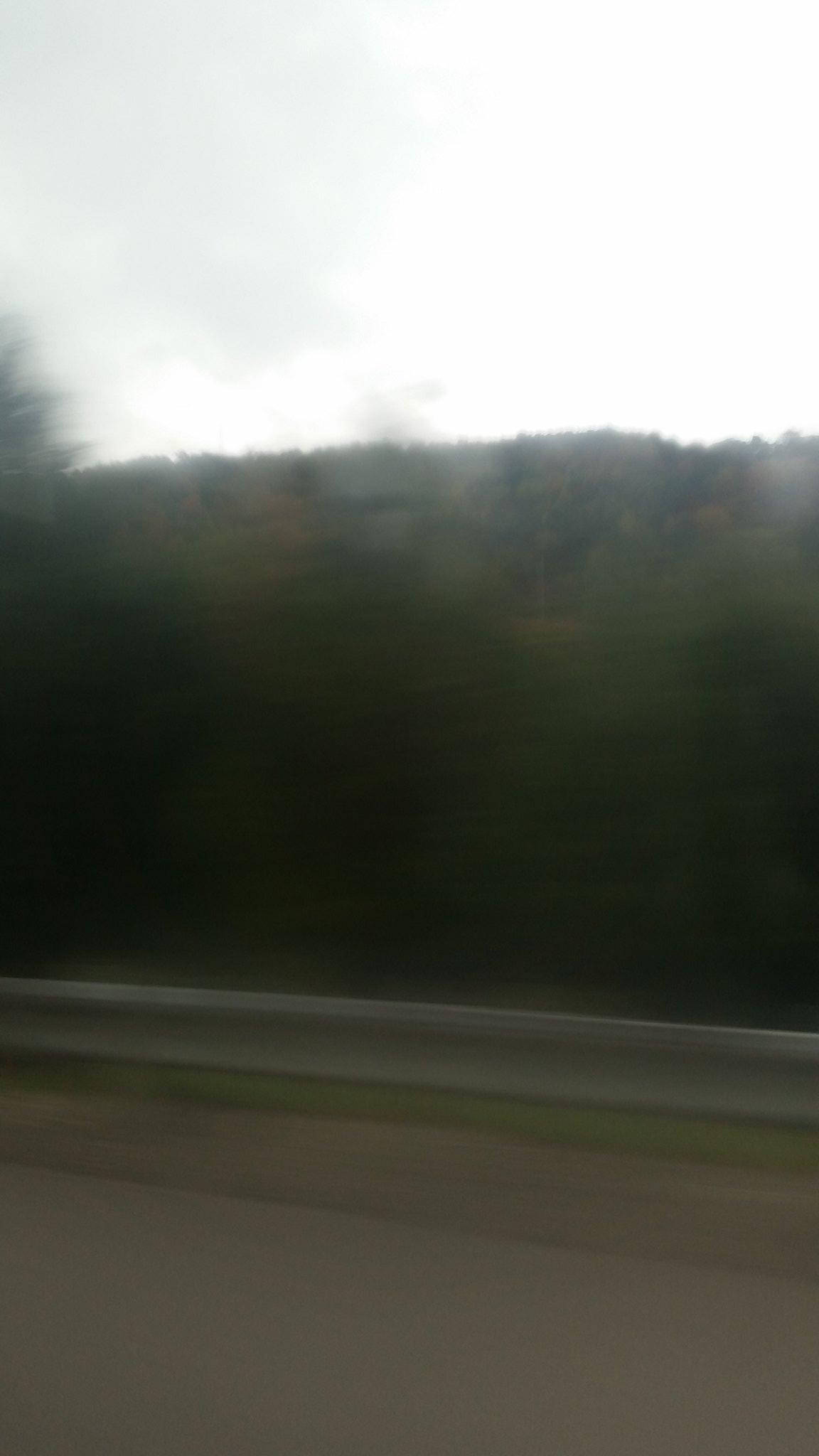A scenic roadway unfolds under a moody sky, suggesting the early moments of sunrise or the closing twilight of sunset. The sky is predominantly covered in dark, brooding clouds, allowing only a hint of sunlight to peek through. The surrounding landscape is lush with verdant green trees, interspersed with patches of leaves tinged with a reddish-orange hue, hinting at the onset of autumn. The road itself is a dark gray cement, exuding a clean, sturdy appearance. A metallic rail runs parallel to the road, serving as a boundary between the pavement and the green grass beyond, adding a sense of order to the picturesque yet somber scene.